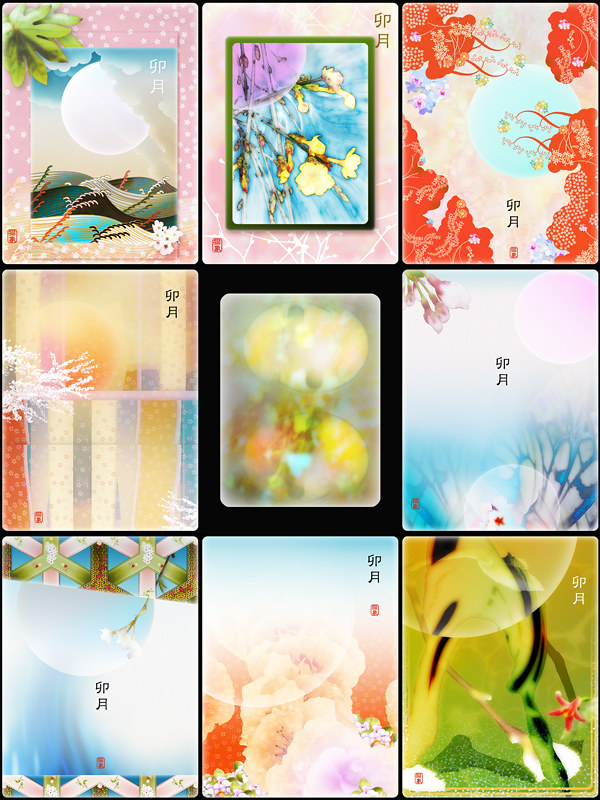This is a collage comprised of nine distinct graphic-rendered images, organized in three rows of three, all encased within a black square border. Each image presents a unique artistic concept:

1. The first image features a pink background adorned with white polka dots. In the corner, green foliage adds a touch of nature. Above, a sun peeks out from behind clouds, and below, blue waves gently roll.
   
2. The second image is bordered in peach and showcases a central object with a green border. The background is blue, decorated with yellow floral-like shapes and a purple moon-like object hovering over the flowers.

3. The third image has a peach backdrop with intricate orange floral details. A light blue moon-like object is positioned in the center, surrounded by blue, pink, and purple flowers.

4. The fourth image displays a series of tan, pink, orange, blue, and yellow lines and shades, interwoven with white. An abstract white tree-like figure overlays this colorful tableau.

5. The fifth image is a somewhat blurry composition bordered in black, featuring an array of green, yellow, white, and blue hues.

6. The sixth image has a light blue background with a central white section. A prominent pink flower takes the spotlight, enhanced by a white lens flare effect.

7. The seventh image, part of the bottom row, depicts a sky-colored background with green and white crisscross designs above and white crisscross patterns below.

8. The eighth image contrasts white with orange, presenting abstract, flower-like figures with hints of purple interspersed throughout.

9. The final image combines green and brown tones, featuring a pink flower. Black lines detail the green object, alongside patches of white, lending the piece a layered, textured feel.

Each image in the collage brings its own unique aesthetic, collectively forming a vibrant and imaginative art piece.